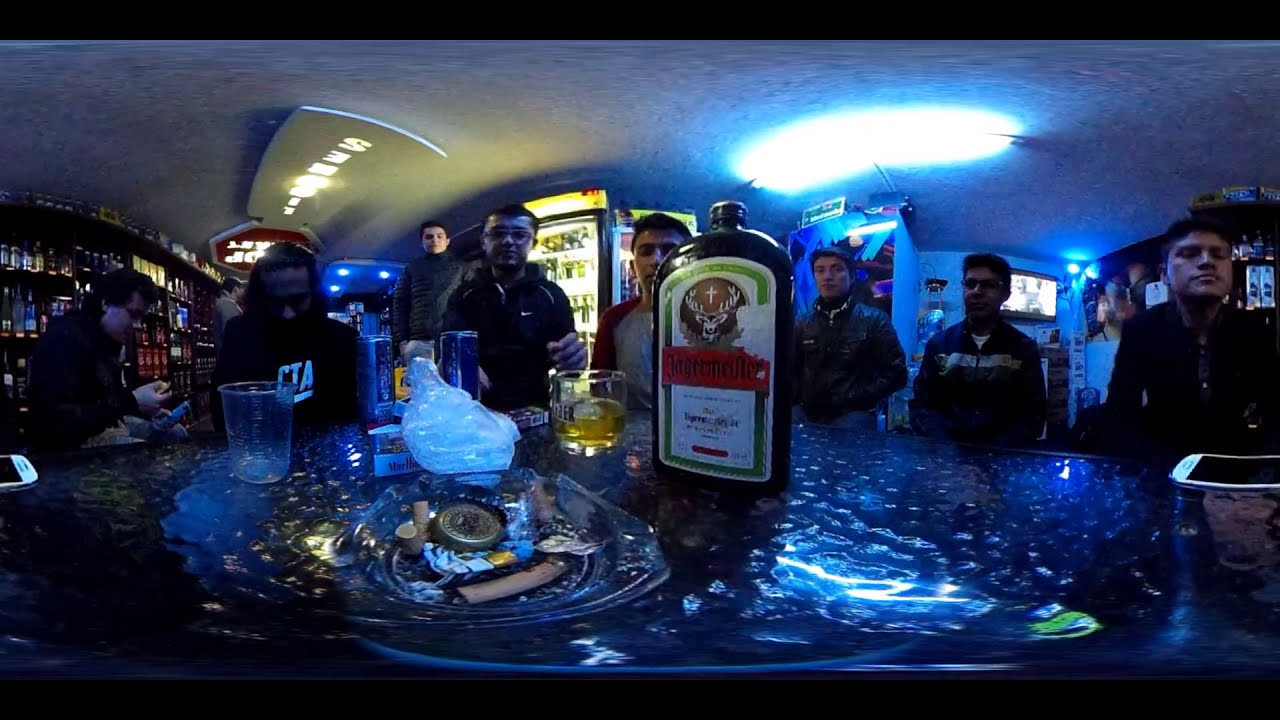The image captures a moody, dark bar setting, characterized by blue ambient lighting and a wide horizontal perspective accentuated by thin black stripes at the top and bottom. Dominating the center is a large, black liquor bottle, identified as Jaeger Meister, featuring a white label with green and red accents, and the iconic deer symbol with antlers of a cross. Surrounding the bottle on the black, dotted counter are an assortment of clear and plastic glasses, an ashtray with cigarette butts, and a phone. A line of nine men dressed in black stand behind the counter, staring directly at the camera. The background reveals an array of liquor bottles displayed on shelves and refrigerators, adding to the bar's lively yet intimate atmosphere.